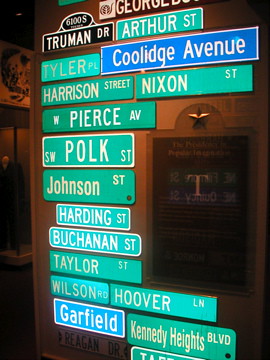This night-time photograph captures an intriguing urban scene featuring a plethora of street signs affixed to the side of a light brown building. The variety of signs, predominantly in shades of green, light blue, and dark blue, each with white lettering, create a visually arresting mosaic. They bear names like Nixon Street, Arthur Street, and Coolidge Avenue, stretching vertically from the bottom to the top of the image.

To the right of this wall adorned with illuminated signs, there's a vertical glass structure, possibly a window or a glass tank, appearing in stark black and contrasting sharply with the lit signs. This setup is located on a street corner, underscored by the moody ambiance of the night. The glow-in-the-dark quality of the street signs adds a distinctive touch, rendering them luminous against the dark background.